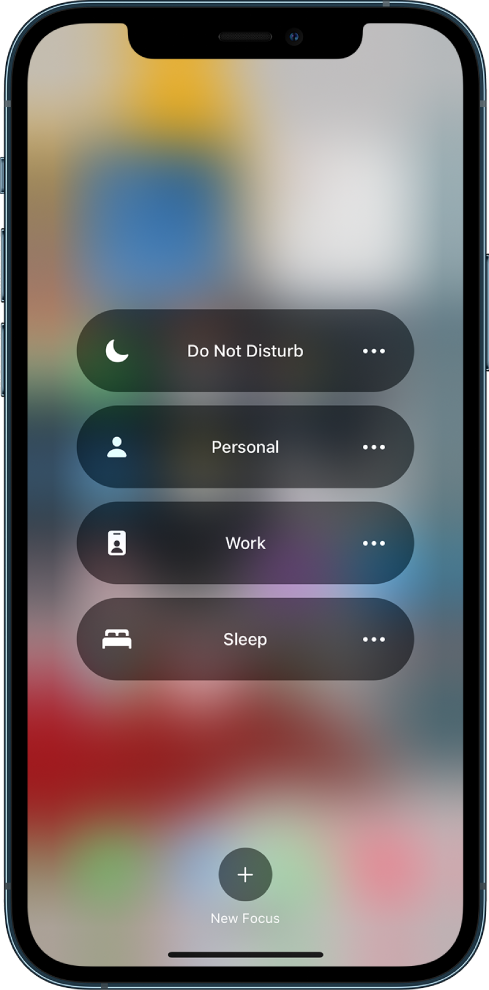This image showcases the Apple iPhone's "Focus" screen designed to help users concentrate by minimizing distractions. The screen displays four elongated, oval buttons against a blurred background, which obscures the iPhone's desktop. Each button is charcoal gray and features white icons and text, along with three ellipsis buttons on the right side for additional options.

Starting from the top, the first button features a moon icon labeled "Do Not Disturb" accompanied by three ellipsis dots. Below this is a button with the icon of a person's profile, labeled "Personal," also with three dots on the right. The third button depicts a white clipboard with a gray person profile icon, and it is labeled "Work," again with three dots on the right. The final button at the bottom displays an icon of a bed and is labeled "Sleep," similarly followed by the three dots for extra options.

At the very bottom, there's a charcoal gray circular button with a plus symbol inside it. Directly underneath this button, white text reads "New Focus," indicating the option to create a custom focus mode.